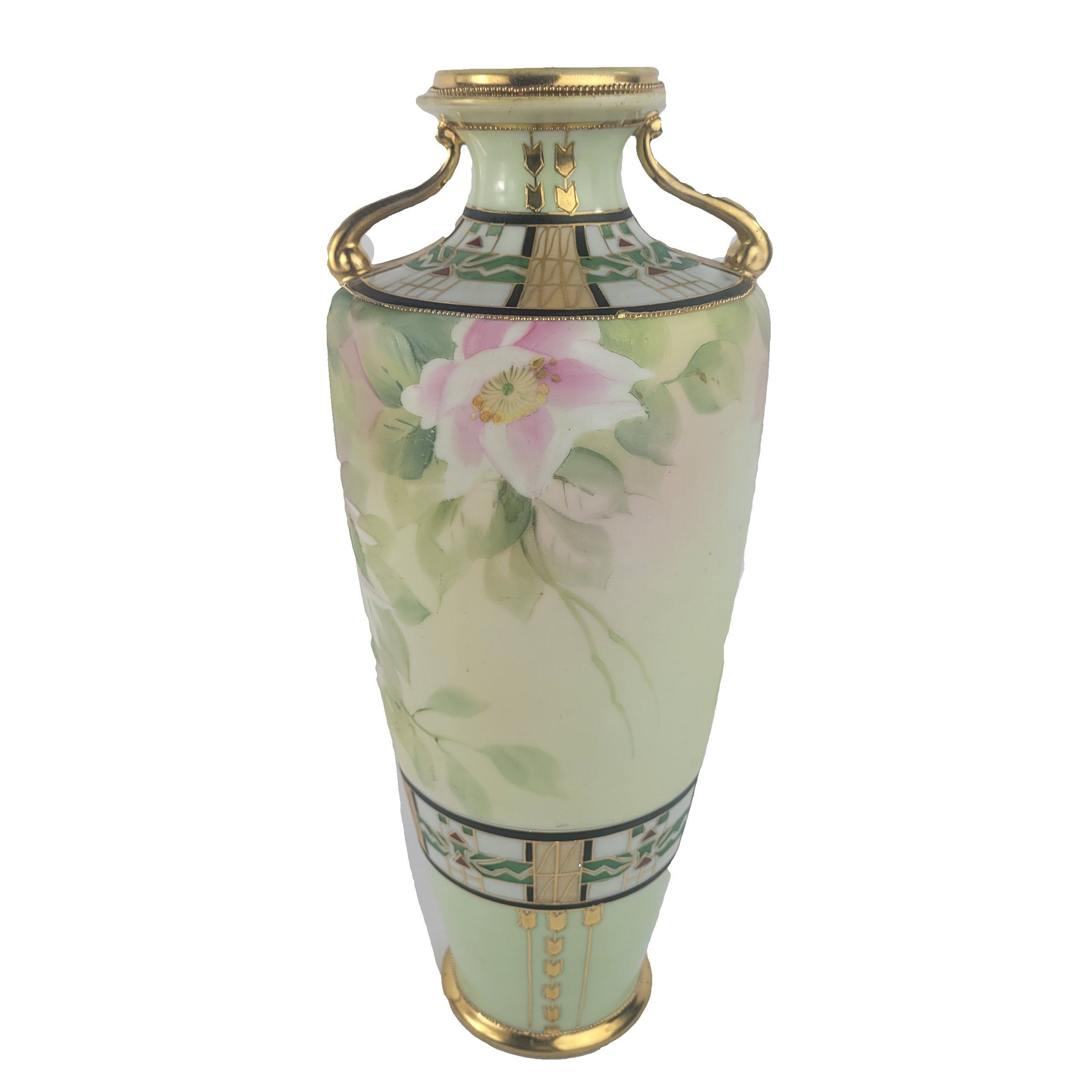This image features a tall, cylindrical, and oriental-style vase, predominantly mint green in color. The vase has a distinctive gold rim at its circular base and another gold rim at the top. It also boasts two elegant, curved gold handles on either side near the top. The centerpiece of the vase's artwork is a striking pink flower with white edges and a yellow center, accompanied by trailing green leaves. The material appears to be a special kind of glass or ceramic, giving it a delicate and ornate appearance, suited more for display than practical use. The background is stark white, making the vase stand out as if it were meticulously placed or even photoshopped into the scene. Additional detailing, such as chevrons in gold, adorns the upper part of the vase, enhancing its intricate and artistic design.